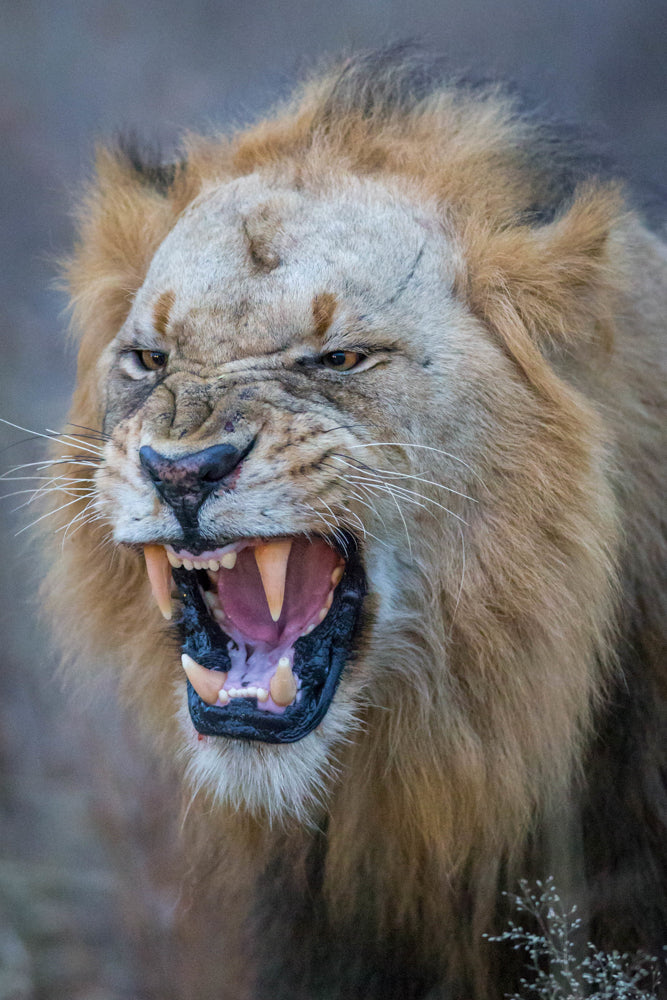This photograph captures a close-up of an aged lion in mid-roar, revealing its powerful presence and intricate details of its facial features. The lion's mouth is wide open, prominently displaying four large, yellowish-orange fangs—two uppers and two lowers—against a backdrop of its tongue. Its heart-shaped, black and wrinkly nose adds to the fierce expression, while white whiskers sprout from either side. The lion's lips are also black, contrasting starkly with the faded, light brown hue of its face. The mane, especially at the top, is notably patchy and light-colored, contributing to the lion's aged appearance. The varying shades of brown on its facial fur range from light to beige, highlighting the lion's majestic yet weathered look. The photograph boasts excellent depth of field, focusing on the lion's snarling face and front coat, which is predominantly a golden or beige color. This detailed image underscores the magnificent yet worn dignity of the king of the jungle.